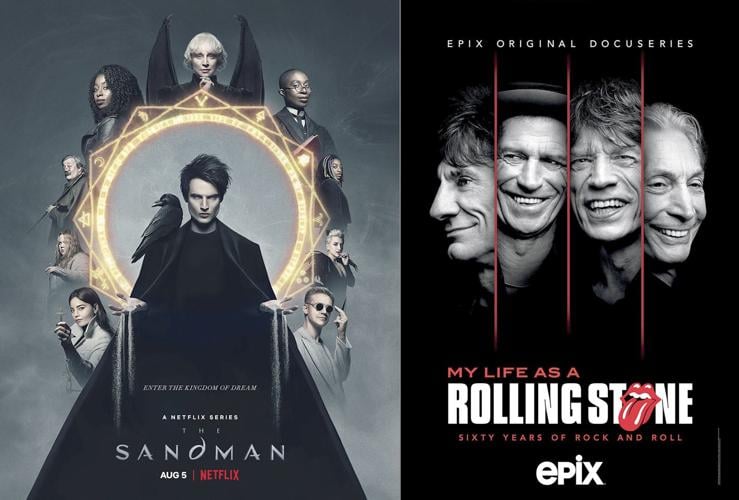The image is a horizontally rectangular poster divided into two vertical sections, each promoting a different show. On the left, a Netflix series titled "The Sandman" is set to be released on August 5th. The focal point is a man in a black trench coat with a raven perched on his right shoulder, who is standing against a gray, smoky background that exudes a mystical atmosphere. Surrounding the man is a geometrical shape, possibly a sphere or sun, with various enigmatic characters encircling it. Above the central figure, there is a black angel. Accompanying the visuals, the text reads "Enter the Kingdom of Dream" in a yellow hue, with "A Netflix Series" and "The Sandman" in white and the release date and "Netflix" in red.

On the right side of the poster, an advertisement for Epix's original docu-series "My Life as a Rolling Stone" features prominently. Set against a completely black background, the top of the image contains the text "Epix Original Docu-series" in white capital letters. Below it, the four black-and-white faces of the Rolling Stones band members are aligned horizontally, divided by thin red lines. Beneath the portraits, the text "My Life as a Rolling Stone" and "60 Years of Rock and Roll" is displayed in white, with the "Epix" logo at the bottom. Red, black, white, gray, gold, and yellow colors are visible across the poster, with red text drawing attention to specific elements.